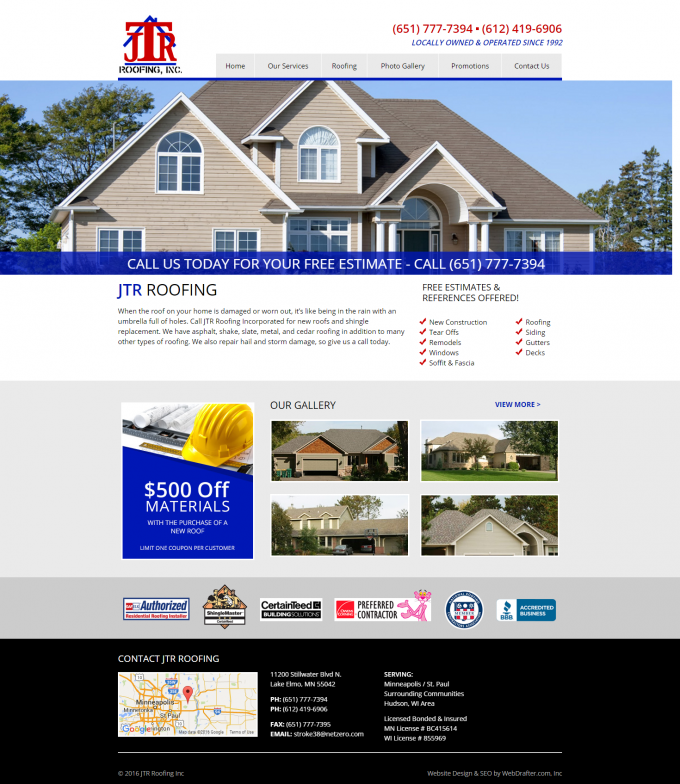This photograph appears to be a screenshot taken from a company's website. The top inch of the image features a white border. About one inch in from the left corner, the company's logo prominently stands out. The logo consists of a bolded "J" and an overlaying, larger "T" that extends over both the "J" and an adjacent "R" on the right. A striking blue line starts from the right of the "R," angles upward above the "T," curves down the left side, and finishes underneath, forming an elegant underline beneath the business name written in black, all-capital letters: "ROOFING, INC."

Below the logo, a long gray navigation bar provides clickable tabs for various sections such as "Contact Us," "Home," and "Services," totaling six different options. Positioned in the top right corner, two phone numbers are displayed side-by-side in red. Underneath these numbers, bold blue capitalized text reads, "LOCALLY OWNED AND OPERATED SINCE 1992."

Dominating the center of the image is a photograph of a two-story house. Framed by a clear blue sky and trees on either side—where the trees on the left are taller and match the house's height—the house exudes an inviting charm. Its light gray façade, punctuated by windows across the front and a partially visible door, stands in contrast to the gray roof. A prominent blue banner stretches across the front of the house with the text: "CALL US TODAY FOR A FREE ESTIMATE – CALL" followed by a phone number. Below this banner, "JTR" is written in blue, followed by "ROOFING" in black.

To the right of the house image, four informational lines detail the company's offerings, mentioning "Free Estimates and References" and their office location. Adjacent to this is a checklist of services featuring five check marks on the left and four on the right.

The lower section of the website features a light-gray border encasing photos of other houses the company has worked on, located on the right side. There is also an image depicting a hard hat and a price. Underneath, six different sponsored labels are displayed. The bottom of the image includes a map accompanied by additional information on the right, all set against a black background.